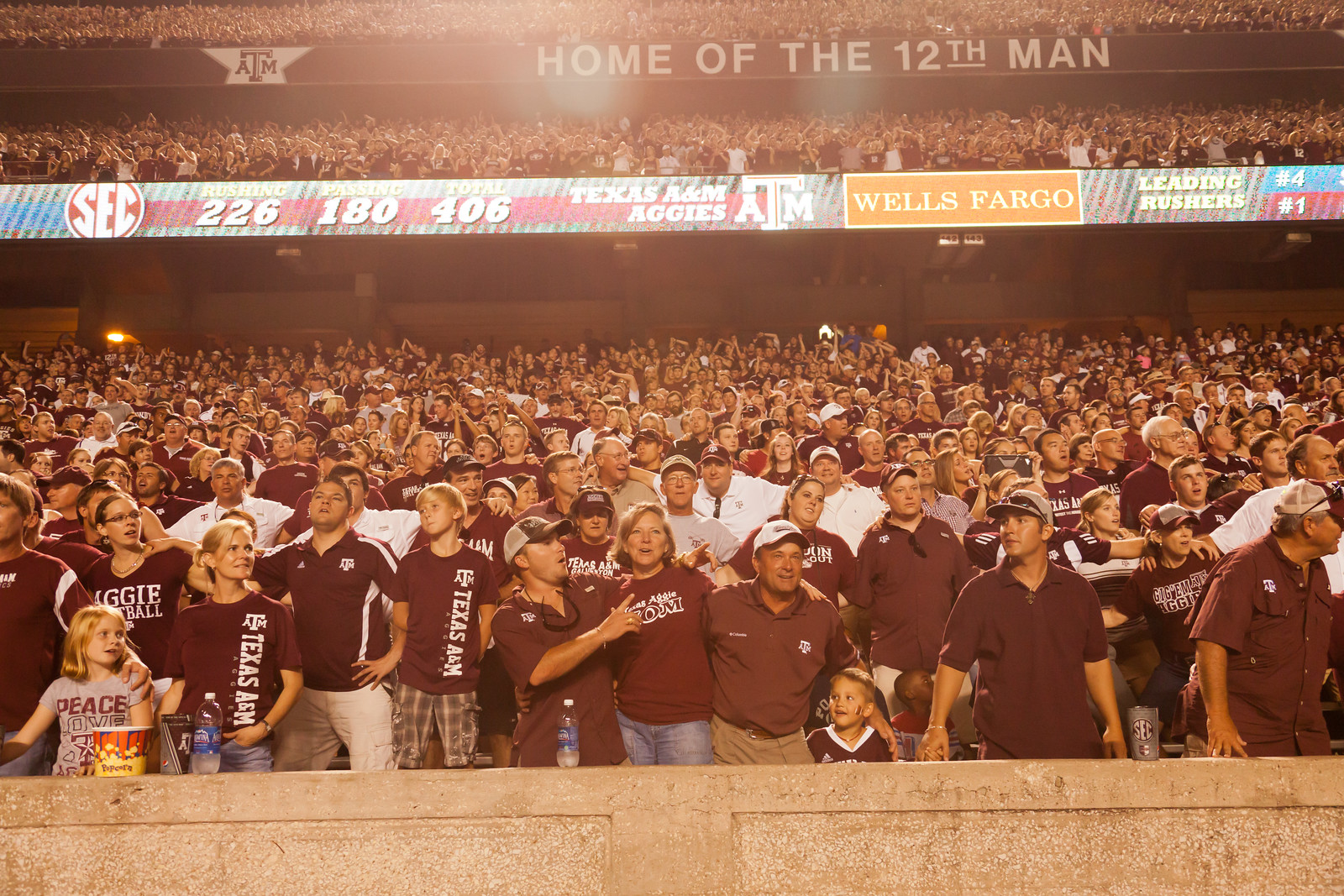A vast and energized crowd of sports fans, predominantly Caucasian and wearing matching brown Texas A&M shirts, fills the stadium bleachers at a sporting event. The photograph captures three tiers of audience members, standing and cascading into the distant rows that extend beyond the lens. Children, women, and men alike contribute to the sea of supporters, underscoring the diverse age range present. In the foreground, a concrete barrier protects the fans from accessing the athlete's area below, featuring a sign with "SEC 226-180-406, Texas A&M Aggies A.M., Wells Fargo." Above this, another sign declares "Home of the 12th Man," indicating Texas A&M's famed tradition. The enormity and density of the crowd, paired with the tiered seating structure, vividly illustrate the stadium's packed and fervent atmosphere.